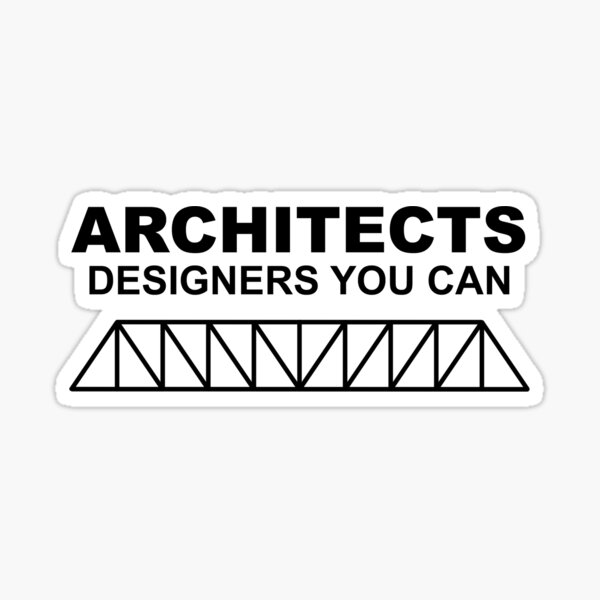The image appears to be a black and white logo or advertisement, likely designed as a sticker for an architect or design firm. It features a solid white background with bold, all-caps black text that reads "ARCHITECTS" at the top. Immediately below that, in a smaller, but still capitalized font, it says "DESIGNERS YOU CAN". Beneath this text, there is a geometric shape, possibly representing a structure or logo. This shape consists of a four-sided figure that is not a perfect rectangle: the top and bottom sides are parallel, but the left and right sides angle outward. Within this shape, there are two large right triangles, pointing inward from each side, and a series of black lines forming zigzags reminiscent of the letter 'N'. These zigzag lines interconnect, creating a dynamic pattern that perhaps represents structural elements or stability, hinting at the idea of trust in professional design and architecture services.